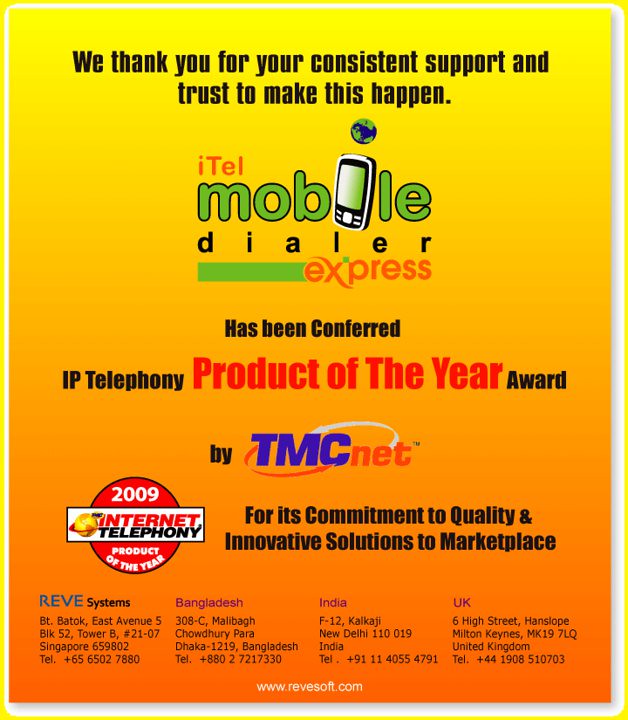This advertisement features a celebratory message and details about ITEL Mobile Dialer Express's recognition as the 2009 Internet Telephony Product of the Year by TMCnet. The top of the advertisement expresses gratitude to users for their consistent support and mentions the award received for commitment to quality and innovative solutions. Visual elements include a background transitioning from bright yellow at the top to orange at the bottom, accented with multi-colored text in orange, black, green, red, purple, and blue. The design incorporates a stylized text where the "i" in "ITEL" is represented by a cell phone with a globe dotting the "i". Another globe, representing the world with green and blue colors, is placed to the left of the text "Internet Telephony." The yellow border and various shades of yellow and orange dominate the advertisement’s color scheme. Additionally, the company’s contact information spans locations in Singapore, Bangladesh, India, and the UK, emphasizing their global presence.